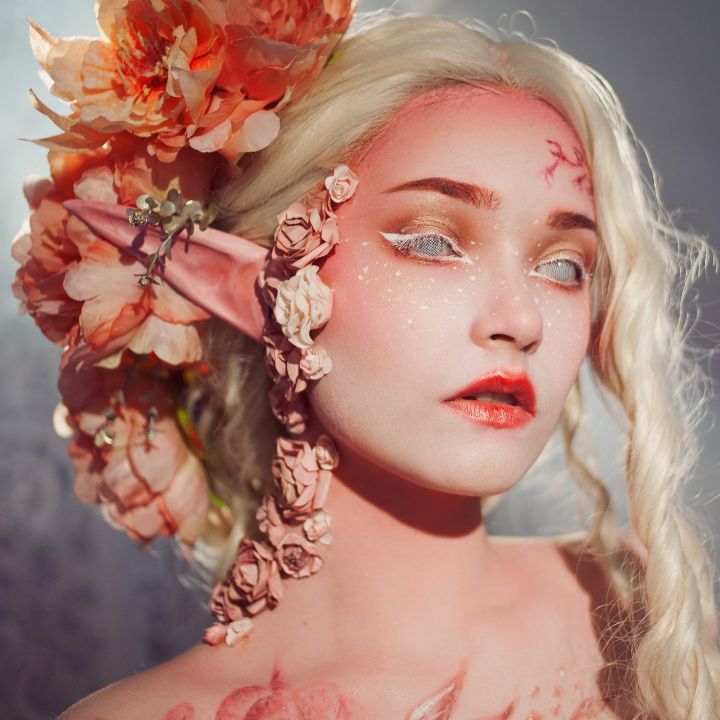This is a highly stylized, color photographic portrait of a young, fair-skinned woman, appearing as a fantasy character. The image, which has a square format, captures her from the top of her head to her shoulders against a digitally created gray backdrop. She faces the right side of the image, with long, whitish-blonde curls cascading around her face on the right, and her hair on the left side tied up into a cornucopia of orange and white flowers that extend from the top of her head to the back of her neck. A separate garland of flesh and cream-colored small roses cascades from her left temple down to her neck.

Her makeup is elaborate, with striking white eyeliner and contact lenses that render her eyes white and cloudy. She accentuates this with white dots on her cheeks and the bridge of her nose. She has dark red lipstick contrasting against her fair complexion. Her forehead features a red, scar-like tattoo on the upper right side of the image. The pointy elf ears, about four to five inches long, add a fantastical element, peeking out prominently from beneath her elaborate floral adornments. 

Her shoulders are bare, revealing peach-colored stenciled designs. The overall photographic style leans towards realism with specialized makeup and accessories creating a fantastical and ethereal effect.